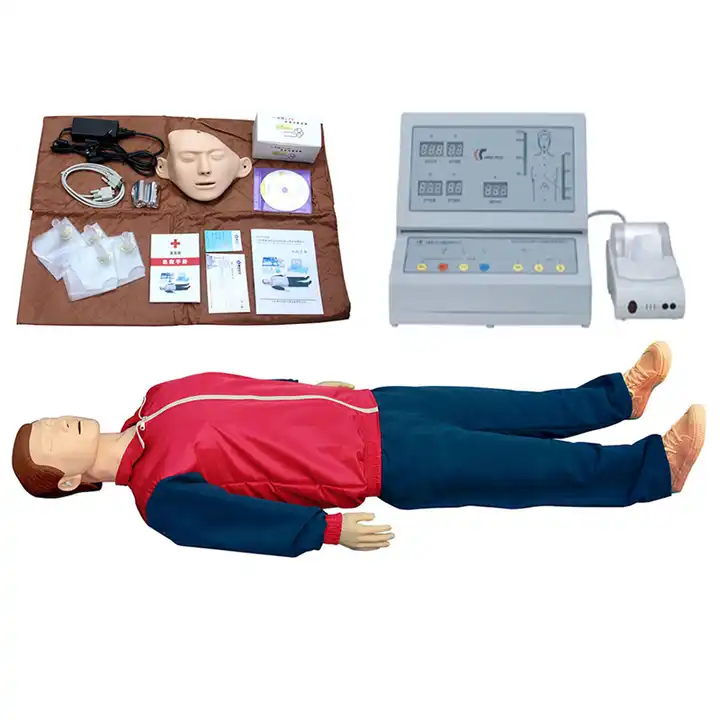This detailed photograph showcases a life-size CPR training dummy dressed in a blue and red tracksuit, specifically wearing blue sweatpants, a red windbreaker jacket with a white zipper, blue sleeves with white trim around the wrists, and off-white sneakers. The dummy has dark blonde to brown hair and lies flat on a brown cloth. Surrounding the dummy are various instructional materials, including brochures, a blood pressure cuff, a face mask, and a DVD. Additionally, there is a rectangular device nearby used to measure vital statistics, featuring a miniature printer presumably for EKG or ECG readings. The machine displays images of the human body with numerical readouts and colorful buttons in yellow, red, white, and blue. A black charger and various cables are also visible, contributing to the array of professional medical training tools.